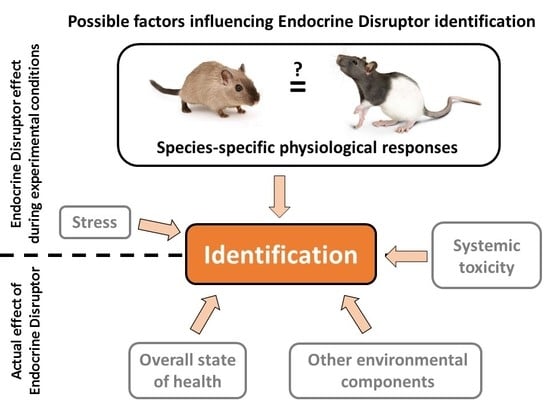The image, likely sourced from a textbook or scientific presentation, is an infographic titled "Possible Factors Influencing Endocrine Disruptor Identification," displayed prominently at the top in black letters. At the center is an orange rectangular box labeled "Identification." Five orange arrows point towards this central box from five surrounding white boxes, each representing different factors. 

The topmost and largest white box features illustrations of two mice, one brown and one black-and-white, separated by an equal sign or possibly an equal sign with a question mark, indicating "Species-Specific Physiological Responses." The remaining four boxes are titled "Systemic Toxicity," "Other Environmental Components," "Overall State of Health," and "Stress." 

On the left side of the image, a dotted line runs vertically. Beside this line, black text reads "Endocrine Disruptor Effect During Experimental Conditions" above the line and "Actual Effect of Endocrine Disruptor" below the line. This detailed and structured infographic highlights various factors and their roles in the identification of endocrine disruptors.